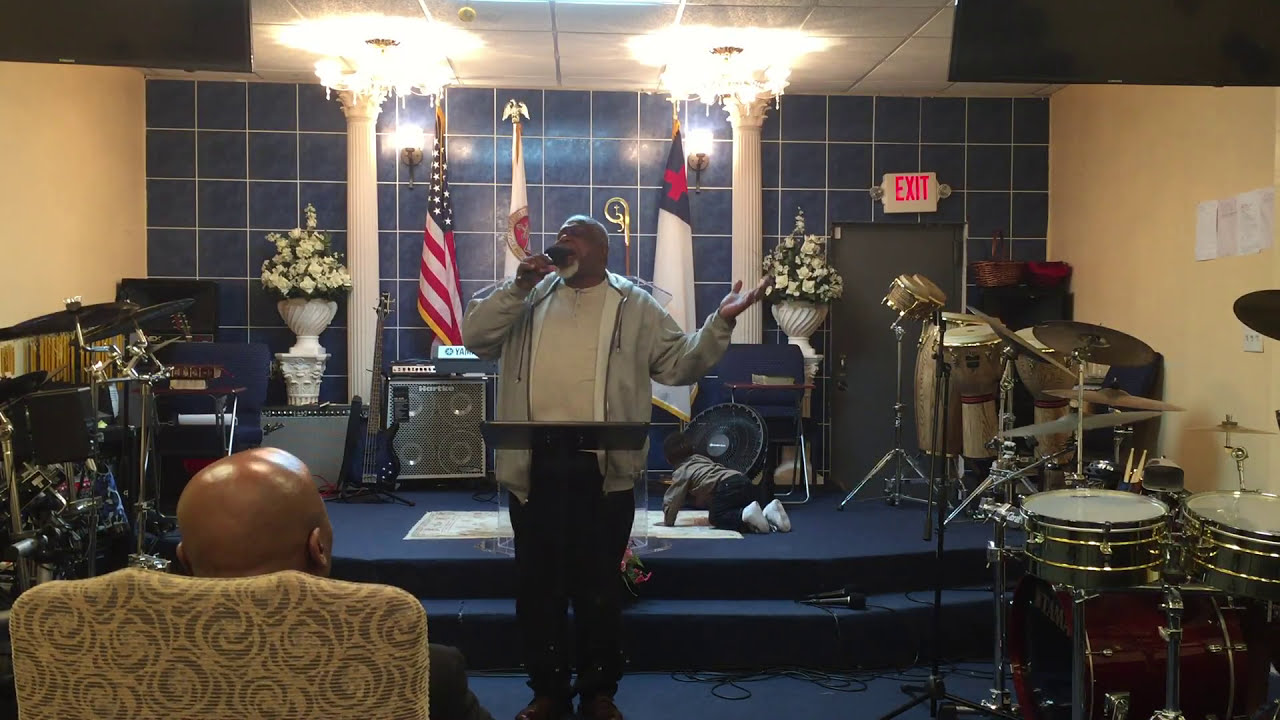In this detailed color photograph, the central subject is an African-American man, standing mid-range at a podium in a small chapel, speaking into a microphone. He wears a gray sweat jacket over a cream-colored shirt and dark pants. The room is adorned with various musical instruments, including a drum set to the right and several guitars possibly standing to the left, alongside speakers and amplifiers. A checkerboard pattern adorns the back wall, which features three flags: the American flag, a white flag with a red cross, and another folded flag. Above the stage are two overhead lighting fixtures.

The podium is situated in front of a multi-layered platform stage, carpeted in dark blue and accessible by two steps. On the stage, a toddler dressed in a gray jacket, blue jeans, and white sneakers crawls on a white blanket, facing away from the camera. The stage is flanked by two white columns, each accompanied by a vase of white flowers and lighting fixtures. There is an exit sign at a doorway to the right.

In the foreground, a bald-headed African-American man is seated with his back to the camera, attentively watching the performance. Additional attendees appear sparse. This image captures a rich, detailed environment, emphasizing both the performer and the intricately decorated chapel setting.